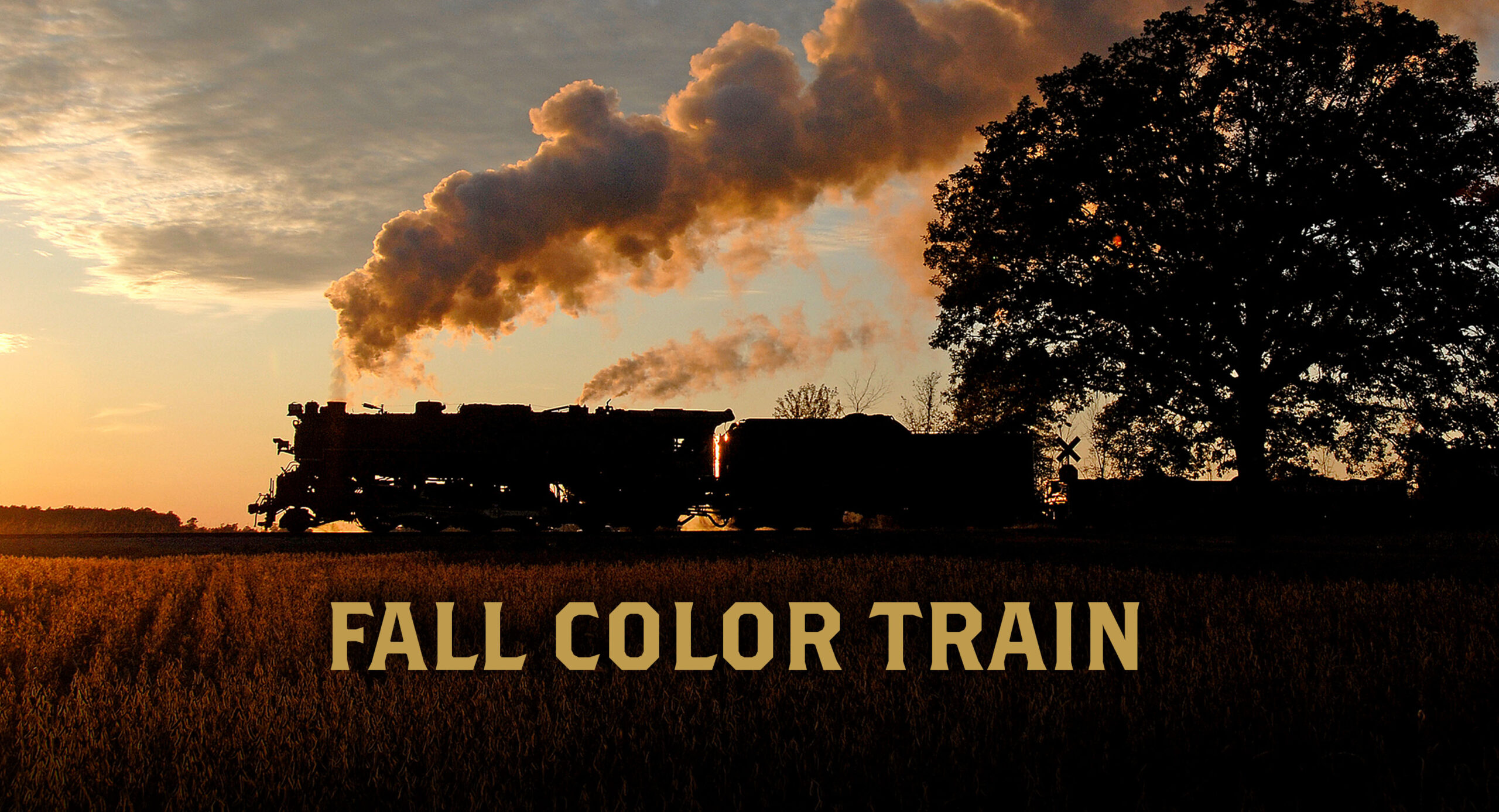This horizontal photograph captures a train traversing a rural scenic landscape at dawn or dusk. The train, moving toward the left, is positioned about halfway down the image and consists of an engine, an enclosed car, and two flatbed cars, with the latter cut off by the image edge on the right. A large, round, leafy tree dominates the upper right portion, silhouetted against the sky due to the lighting. A massive billow of dark gray smoke, edged with a golden vapor, emerges from the train's front engine and drifts to the right. The backdrop reveals a partly cloudy sky with sunlight emanating from the left, casting a glow that illuminates a field of wheat in the foreground.